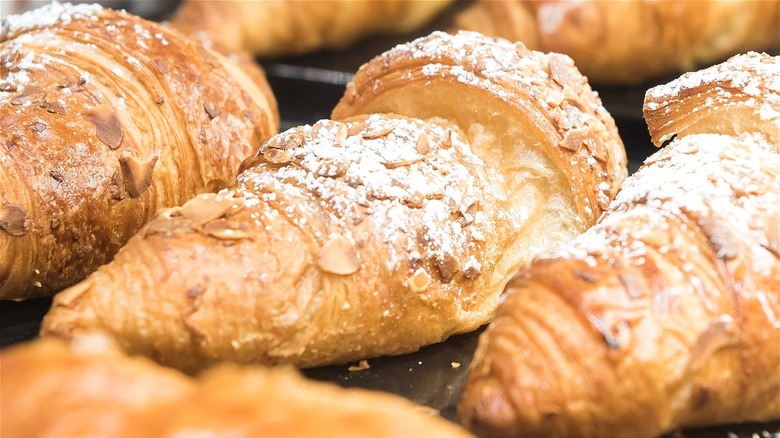This color photograph is an extreme close-up of almond croissants. The image prominently features three croissants in clear focus, with three additional croissants blurred in the background—two at the top and one at the bottom. The croissants have a light, golden-brown hue, adorned with toasted almond slivers and a fine dusting of powdered sugar. The middle croissant is the clearest, while the one on the right is slightly darker and less sharp. All the croissants sit on a dark metal tray, emphasizing their freshly baked, fluffy texture. The background is devoid of any text, people, animals, or man-made structures.